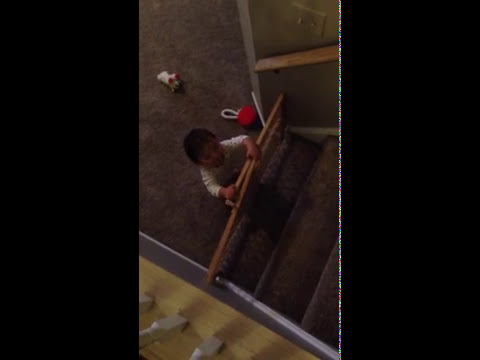The photo, taken indoors from a downward angle, captures a young child with dark skin and black hair standing near the foot of carpeted stairs. A child safety gate blocks access to the stairs, preventing the child from going up. The carpet, like the rest of the area, is brown. The child stands with hands gripping the railing, looking upward. Close to the child, on the dark, carpeted floor, lies a red and white toy, albeit somewhat blurry. The background of the image features an empty bookcase. Additional objects in the scene include visible rails on the bottom left, toys scattered on the floor, and a light switch in the upper right corner. The child is centrally positioned in this photograph, which might be part of a triptych, indicated by the black left and right panels bordering the central image. The overall setting appears to be possibly a basement area of a house, though the exact lighting conditions are unclear.